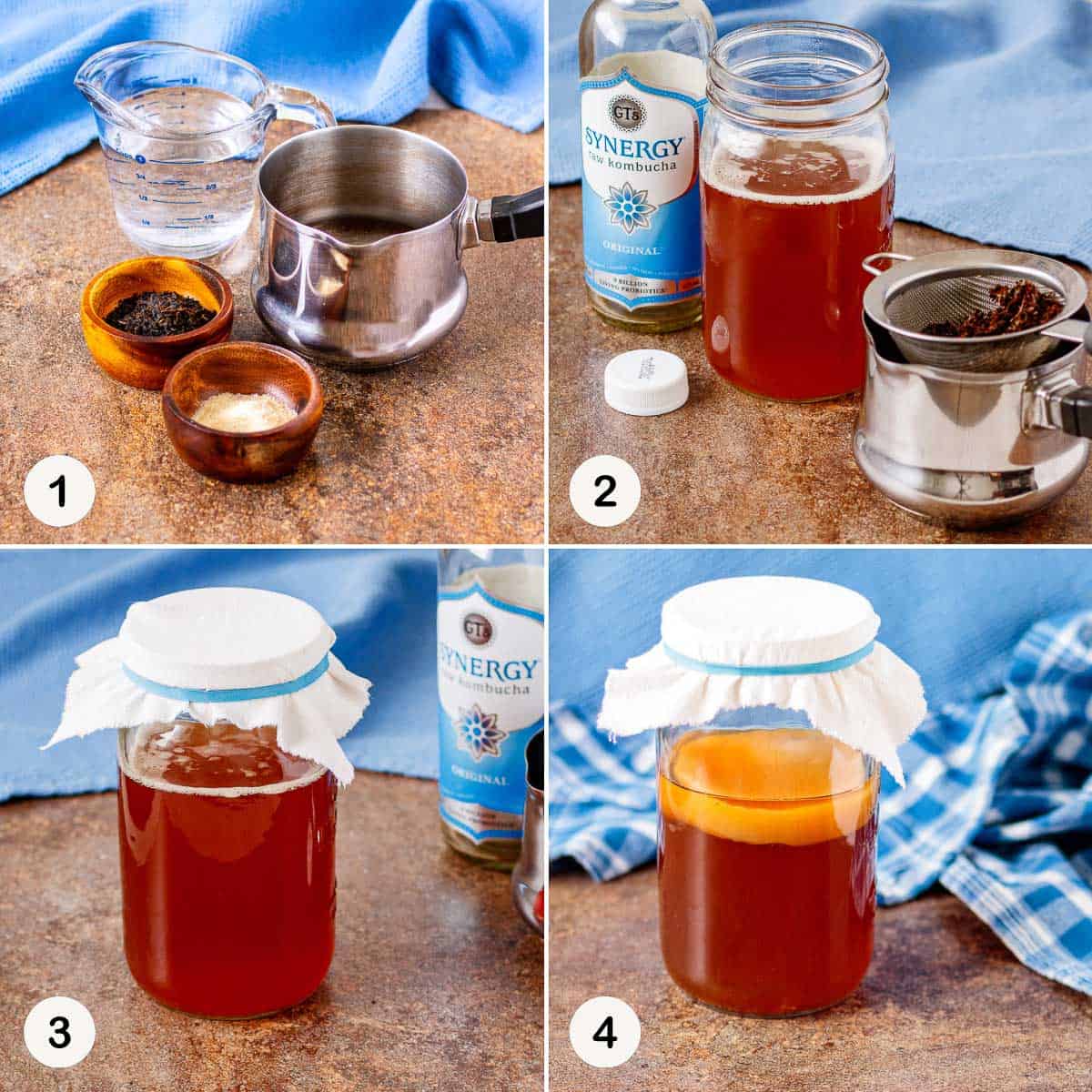This instructional image showcases a step-by-step guide for brewing kombucha, divided into four equally cut squares labeled 1, 2, 3, and 4. In the first square, labeled number 1 at the top left, a small pot with a silver lip is visible on the right side, accompanied by a wood grain bowl containing white powder at the bottom and another yellow wood grain bowl with black seeds above and to the left. A liquid measuring cup filled with water with blue markings can be seen at the top. A photograph completes this image, and a white circle with black text marks the bottom left. 

The second square, labeled number 2 at the top right, displays a mason jar filled with amber liquid. A GT's Synergy Raw Kombucha bottle with a blue label and white cap is seen at the top left, while a pot containing a tea infuser with leaves sits below, emphasizing the brewing process.

In the third square, labeled number 3 at the bottom left, the same mason jar now covered with a white cloth secured by a blue rubber band indicates the fermentation process. The GT's Synergy bottle appears in the background.

Finally, the fourth square, labeled number 4 at the bottom right, shows the completed kombucha. The mason jar with a white cap reveals yellow foam on top of the liquid, against a backdrop of a blue plaid blanket, signifying the finished brew ready for consumption.